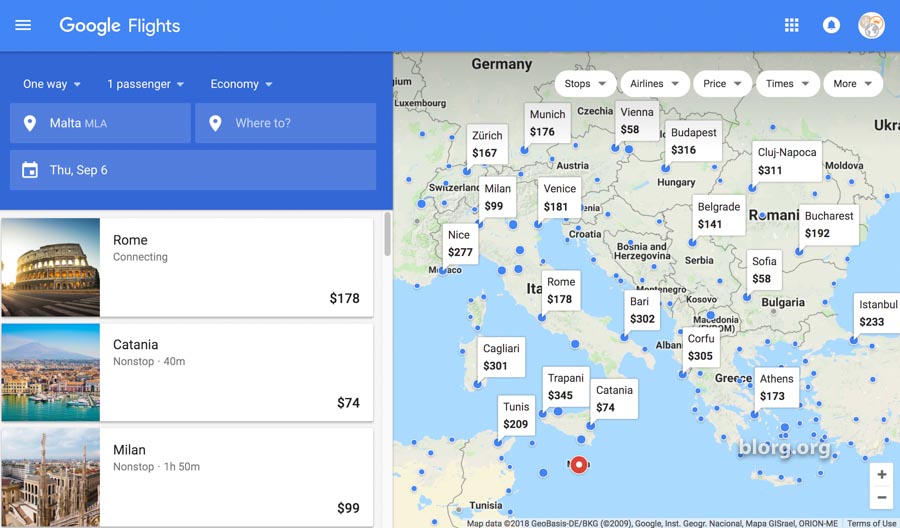This is a detailed screenshot of the Google Flights interface centered on a map of Eastern Europe, stretching from Italy to Ukraine. At the top of the screen, a blue navigation bar displays "Google Flights" along with options for menu access, notifications, and profile settings. 

On the left side, flight details for a one-way trip in economy class for one passenger departing from Malta are provided, with the destination field left open. The selected departure date is Thursday, September 6th. These details are highlighted in a darker blue box. Below this box, a white, scrollable pane showcases potential destinations: Rome, Catania, and Milan, each accompanied by an image of iconic architecture.

To the right, the map section features approximately 50 blue dots indicating various cities, with around 15 of these dots accompanied by message boxes detailing the city name and flight costs, which range from $58 to $302. Beneath the map, there are white filter options that allow users to refine their search by stops, airlines, price ranges, departure and arrival times, among other criteria.